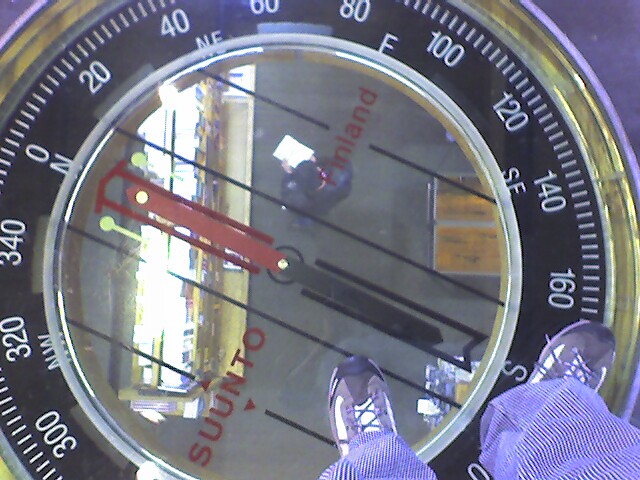This photograph captures a unique perspective of an individual standing on a large, round navigational instrument, likely a compass. Visible in the image are a pair of feet clad in gray, black, and white sneakers with laces, standing on the device. The person is wearing white or blue and white striped pants. 

The compass features a white border encircling a ring of bright, brassy color. Within this brassy ring is a black circular section adorned with markings that resemble those on a compass. Starting at the top, oriented towards 0 and N, the markings progress in increments of 20 degrees: 20, 40, NE (Northeast), 60, 80, E (East), 100, 120, SE (Southeast), 140, 160, S (South)—with the S located near the right foot. The sequence continues further around the circle: 300, 320, NW (Northwest), 340. Between these prominent numerical indicators are smaller white hash marks denoting individual degrees.

The reflective face of the compass has a needle, which is half black and half red, pointing within the device. The reflection on the compass face is indistinct, adding a sense of mystery to the image. Adorning the face of the compass are red letters spelling out "SUUNTO" and additional black lines, along with the word "Finland" in red on the right side.

The overall image intricately details both the design and function of the compass, emphasizing its utility and craftsmanship.